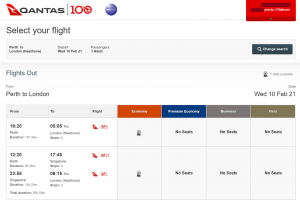The image appears to be a screenshot from the Qantas website, specifically the page where users can select their flights. The Qantas logo, featuring a stylized red tail fin with a distinctive white silhouette, is prominently displayed in the upper left corner. The headline "Select Your Flight" indicates that this page is for choosing flights, specifically from Perth, Australia to London, England.

Displayed on the page are several flight options with different departure times from Perth to London for the selected date, Wednesday, 10 February 2021. The flight details such as departure and arrival times, as well as prices, although present, are too small to be legibly read in the image.

In the upper right corner of the page, there is a red rectangular area with text that has been obscured or crossed out, making it difficult to decipher its contents. Below this red rectangle, there is a blue search button marked with a magnifying glass icon, indicating functionality for flight searches or modifications.

The overall layout includes a detailed interface for users to review and select their preferred flights, though the finer details of each flight option remain indistinguishable due to the small text size in the image.